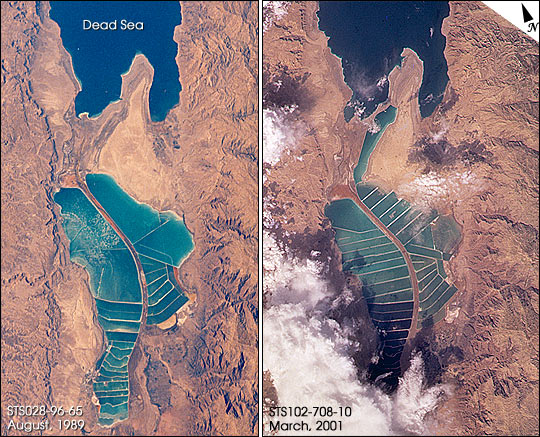In this detailed aerial image, we see two side-by-side high-vantage point shots showcasing the same geographic location at different times. Both images feature a landscape dominated by the brown, rocky terrain characteristic of areas surrounding the Dead Sea. The photograph on the left, labeled "STS 028-96-65 August 1989," presents the irregularly shaped, blue-colored waters of the Dead Sea, prominently outlined and labeled in white text at the top. The land flanking the Dead Sea retains a relatively uniform, rugged appearance.

The right-hand photograph, although identical in orientation, is dated "STS 102-708-10 March 2001." It conspicuously lacks the text labeling the Dead Sea and shows the body of water in black instead. A notable difference is visible in the lower left corner, where a white covering—potentially clouds or snow—appears, overlaying part of the landscape. This white covering partially obscures the mountainous terrain below. Additionally, the land between the mountain ranges in the valley area appears to be more partitioned, suggesting possible land use changes over the intervening years. Together, these images offer a comparative visual study of geographical transformations around the Dead Sea over a span of more than a decade.